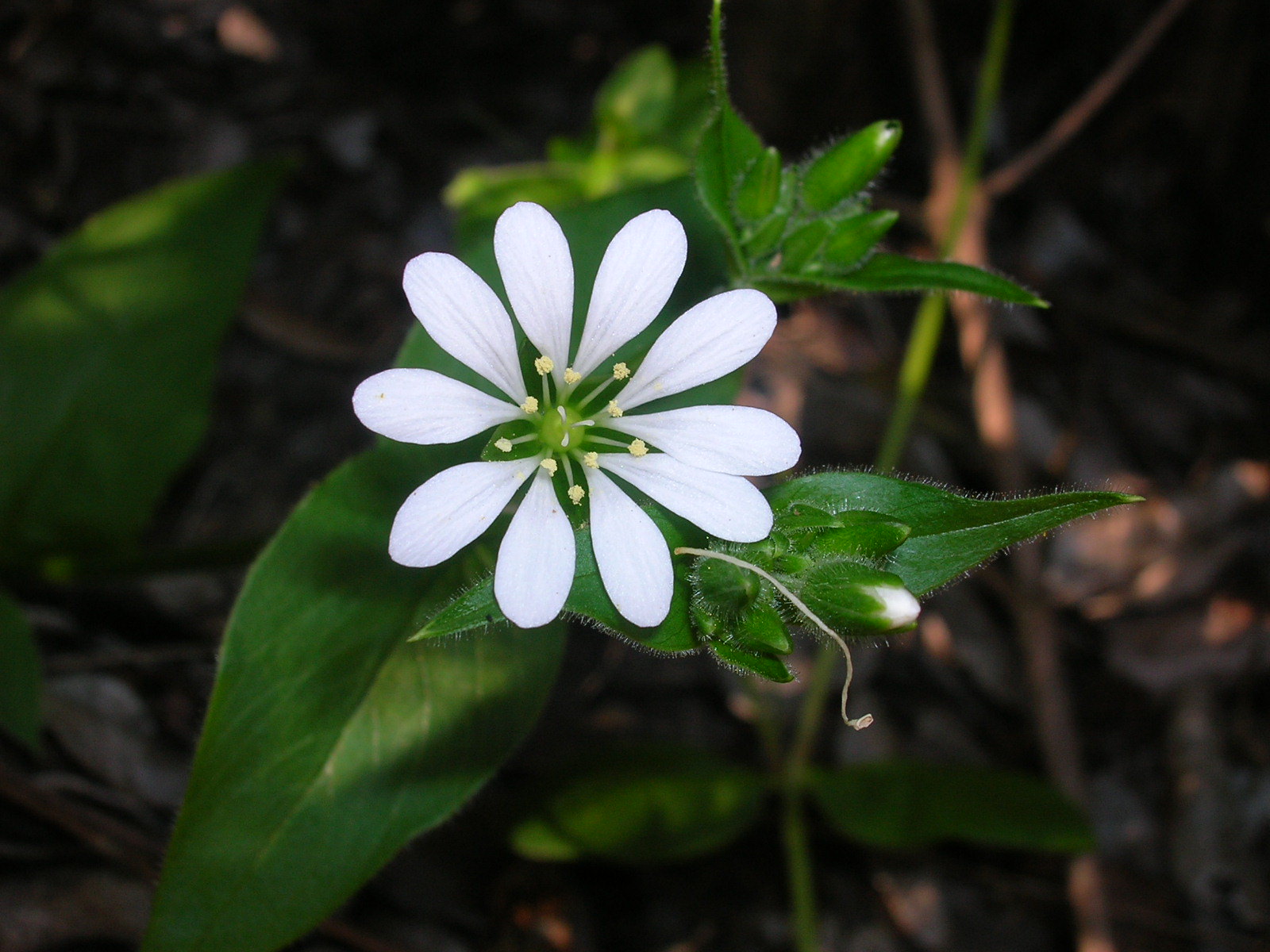This is an outdoor photograph of a vibrant white-petaled flower with green leaves. The plant is situated on a forest floor scattered with dead leaves and wooden debris, which are various shades of brown. The flower boasts nine to ten distinct, paddle-shaped petals arranged in a sun pattern around its center. This center is a cluster of small, yellow, popcorn-like kernels attached to green stems. The flower is attached to a green stem, with some of the foliage displaying fine hairs. Additionally, there are budding flowers still encased in dark green pods. The leaves exhibit a gradient from dark to light green, depending on how the light hits them.